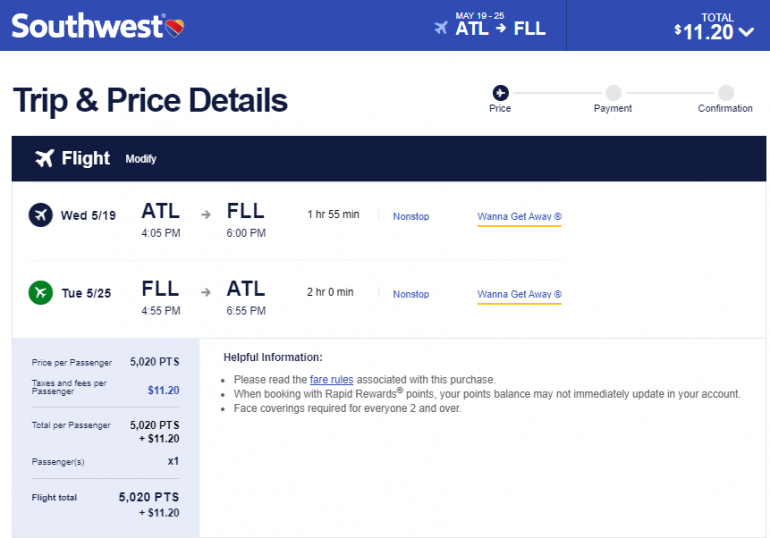### Descriptive Caption for a Southwest Airlines Booking Screenshot

This screenshot captures a Southwest Airlines flight booking on a smartphone interface. At the top, the familiar Southwest Airlines logo is displayed, followed by the text "May 19th through 25th." An airplane icon links Atlanta (ATL) with Fort Lauderdale (FLL), indicating a round-trip journey. To the right, the total fare is displayed as $11.20 with a dropdown arrow.

Beneath this section, a white box labeled "Trip and Price Details" is prominently featured. Below it, a progress bar with three steps— "Price," "Payment," and "Confirmation"—shows the current booking phase, with "Payment" highlighted in a gray circle.

A black section follows, containing an airplane icon next to the word "Flight." The flight details are listed below, starting with the outbound flight: 
- **Wednesday, May 19th**
  - Departs ATL at 4:05 PM
  - Arrives FLL at 6:00 PM
  - Duration: 1 hour 55 minutes
  - Marked as "Nonstop" under the "Wanna Get Away®" fare category

The return flight details are next:
- **Tuesday, May 25th**
  - Departs FLL at 4:55 PM
  - Arrives ATL at 6:55 PM
  - Duration: 2 hours
  - Also marked as "Nonstop" under the "Wanna Get Away®" fare category
  - The cost per passenger is listed as 5,020 points

Additional helpful information is found below these details, including important note points such as:
- "Please read the fare rules associated with this purchase."
- "When booking with Rapid Rewards points, your points balance may not immediately update in your account."
- "Face coverings are required for everyone aged 2 and over."

This organized and informative layout ensures passengers have all the necessary details for their upcoming trip with Southwest Airlines.